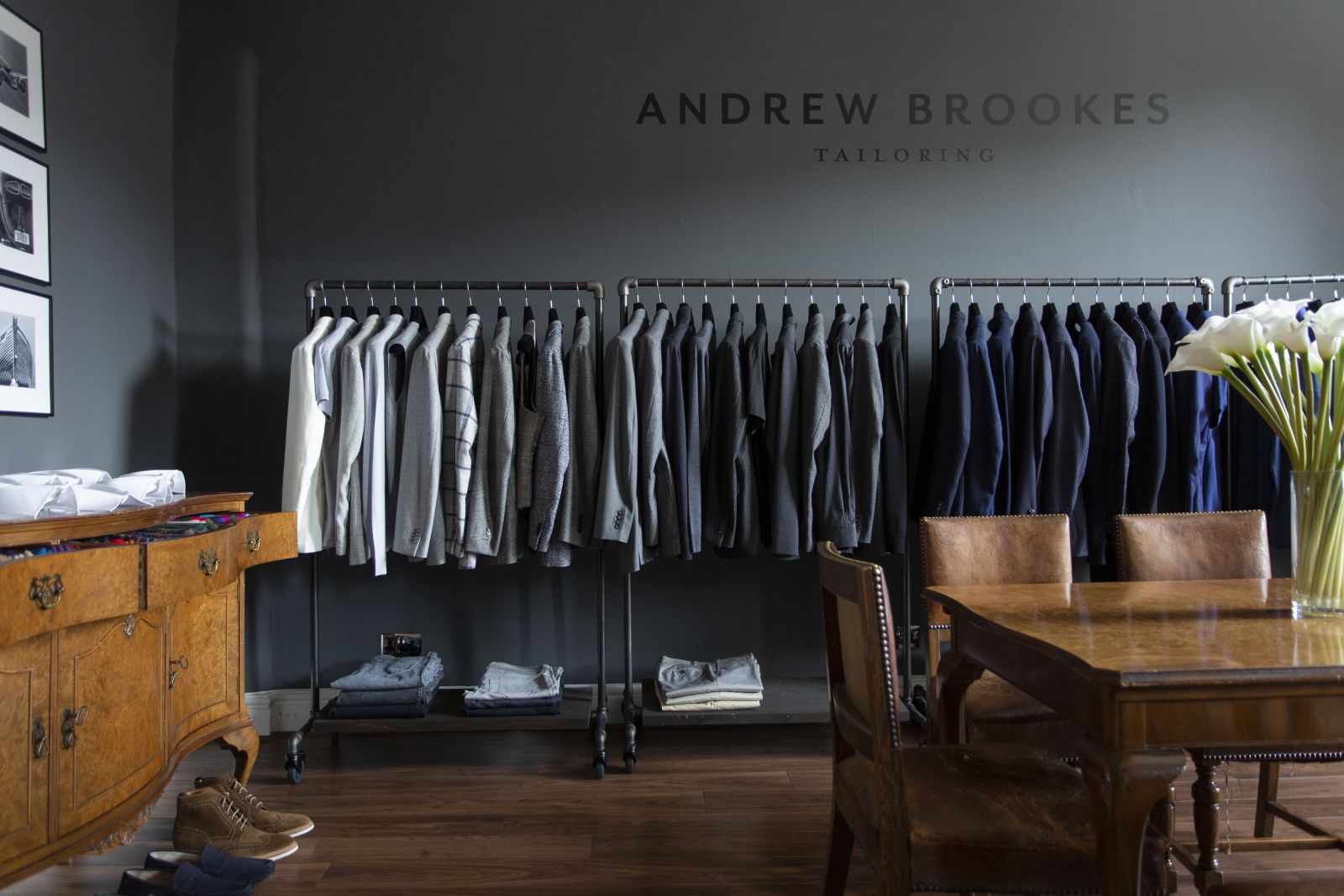The image showcases the interior of Andrew Brooks Tailoring, painted in a dark gray hue. Prominently displayed on the wall is a sign reading "Andrew Brooks Tailoring" in all caps, with "tailoring" in smaller font, set against the light gray background. Beneath this sign, a series of four clothing racks on wheels hold a collection of neatly hung shirts and jackets in an array of subdued tones such as white, gray, dark blue, and black. Below these hanging garments, folded shirts rest on a lower shelf integrated into the racks. 

To the left, an armoire with three large drawers, which appear to contain ties, and three cabinets underneath sits against the wall. On top of this armoire lies a neatly folded white shirt. Framed photographs in black frames are aligned vertically to the left of the armoire. On the floor before it are two pairs of shoes—a black pair and brown ankle boots. 

To the lower right corner of the image, a sophisticated brown wooden table with three leather-backed chairs is positioned. Adorning the center of the table is a clear glass vase filled with white flowers, possibly lilies. The room exudes a refined and orderly ambiance characteristic of a high-end tailoring shop.